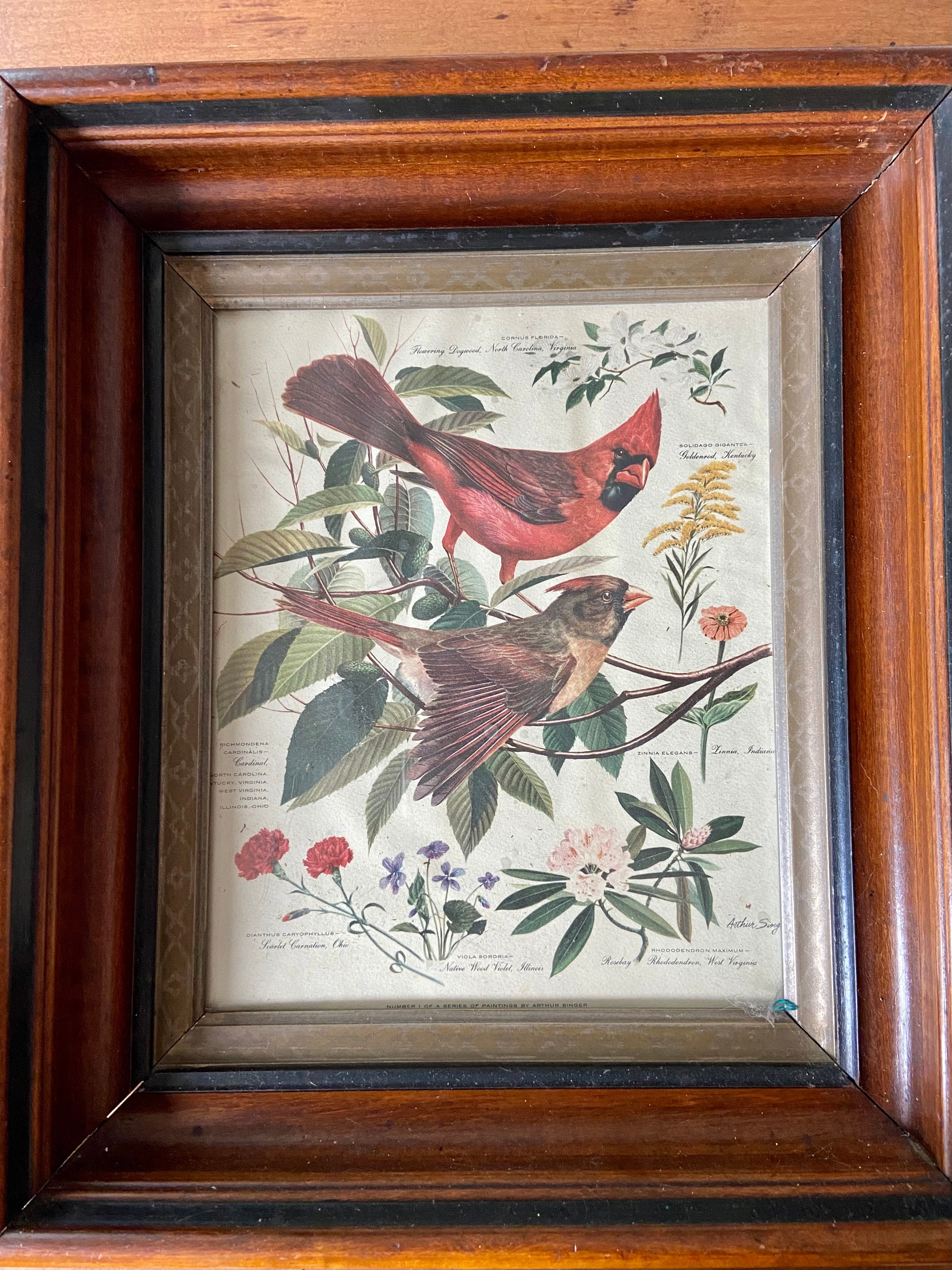This is a color photograph depicting an ornately framed, aged botanical print. The thick wooden frame features a detailed color scheme consisting of silver, black, dark brown, and light brown bands, lending a distinguished appearance to the piece. The print within exudes an air of antiquity with its slightly dusty, off-white background. The illustration, however, is remarkably vivid, showcasing two birds perched on a slender branch with leaves. The top bird appears to be a cardinal, characterized by its bright red plumage and black facial markings, while the lower bird boasts a mix of dark brown and light brown feathers with a distinct yellowish-orange beak and red tail. Surrounding these birds are a variety of flowers, including roses to the left and purple blossoms next to white lilies towards the right, reminiscent of a scientific botanical illustration. Despite the old print, the names of the flowers remain legible. This elegant and detailed depiction captures the natural beauty and delicate interplay of flora and fauna.